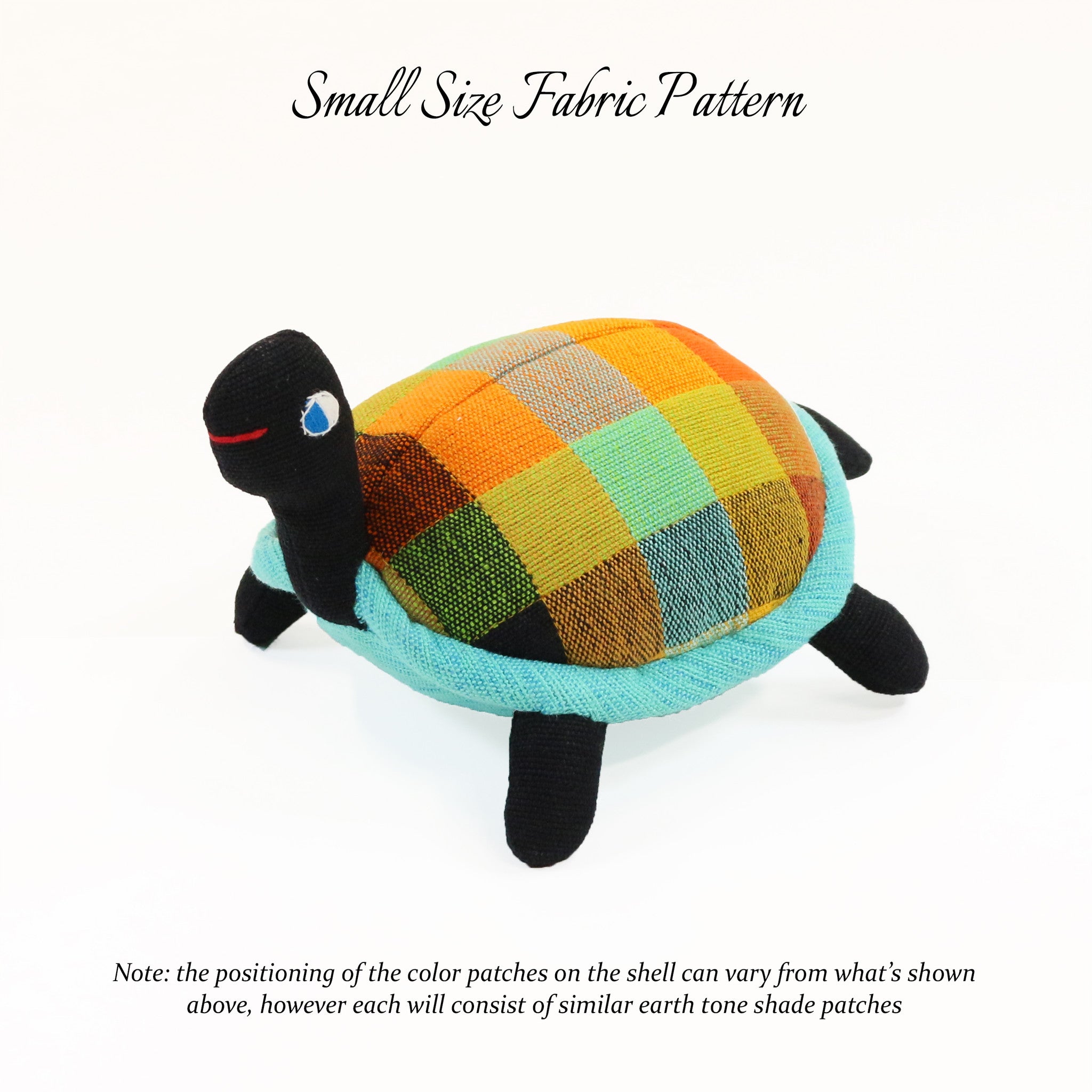The image showcases a charming plush turtle against a blank white background. The turtle features a textured shell made from fabric with an intricate patchwork checkerboard pattern in various earth tones, including shades of orange and yellow. Each shell might vary slightly in the positioning of patches but retains similar color schemes. The shell is bordered by a light blue fuzzy fabric, adding a touch of softness to its appearance. The turtle’s body parts, including the head, limbs, and tail, are solid black. Its face is designed with simple blue eyes that have a white outline, and a red line forms its mouth, giving it a playful, human-like expression. Above the turtle, there is a title that reads "Small Size Fabric Pattern", and beneath the turtle, there are two lines of smaller text that provide further details, including a note that the positioning of the color patches on the shell can vary.